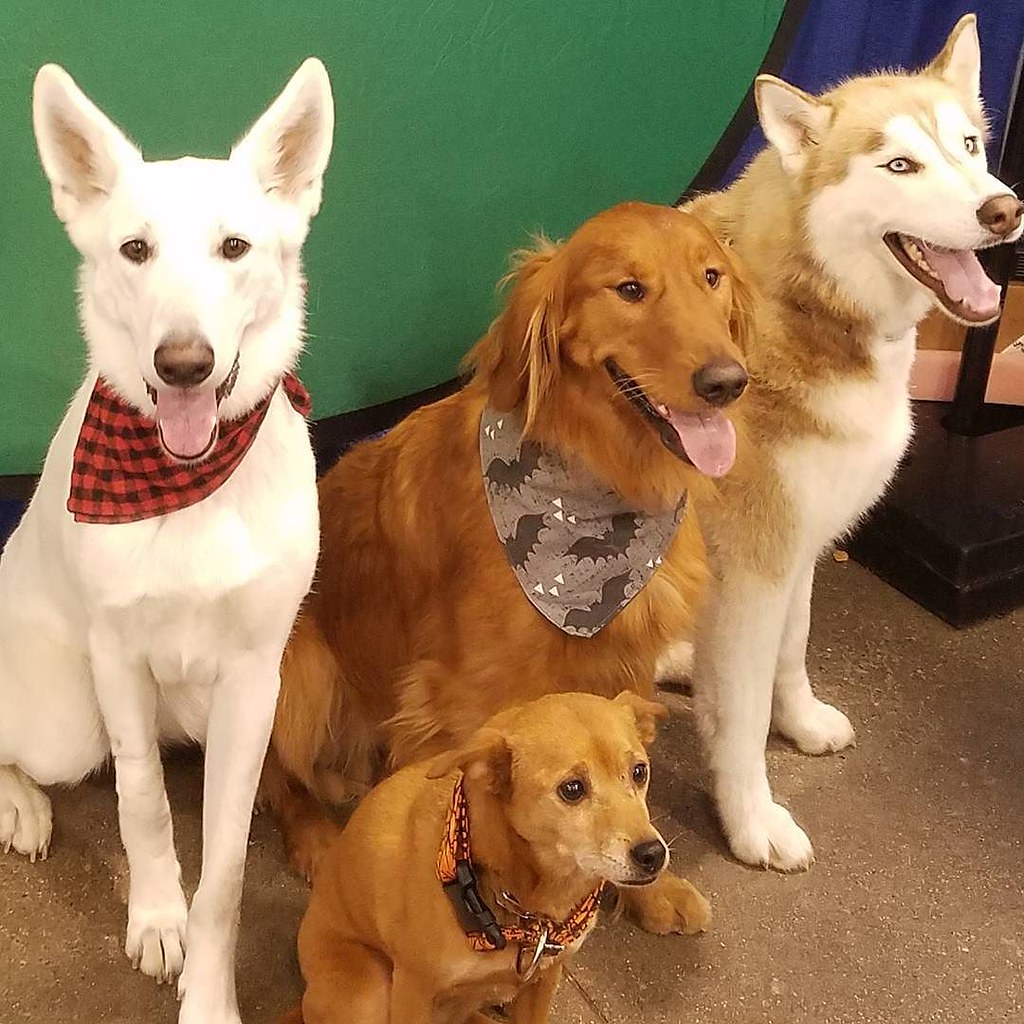In this detailed photograph, four dogs are sitting closely together inside a room, exuding a sense of camaraderie and charm. Foremost on the left is a white dog with perky ears adorned in a stylish red and black crisscross checkered handkerchief. Next to him, slightly in front, is a smaller, mid-brown dog, notable for his orange collar and floppy ears. Positioned alongside is an elegantly fluffy golden retriever sporting a bat-themed neck scarf, his golden fur framing his face with a semi-serious expression. Completing the quartet, the rightmost dog, resembling a husky, boasts striking lighter-colored eyes and a mix of white and coppery fur. While the three larger dogs express enthusiasm with open mouths and visible tongues, the smaller dog's mouth remains closed. Their different gazes reflect the scenario of multiple people capturing the moment, capturing the dogs' attention in various directions. The backdrop of the image reveals a green background with a hint of blue off to the side, and they are all perched on a grayish-brown surface, adding to the cozy and informal vibe of the scene.